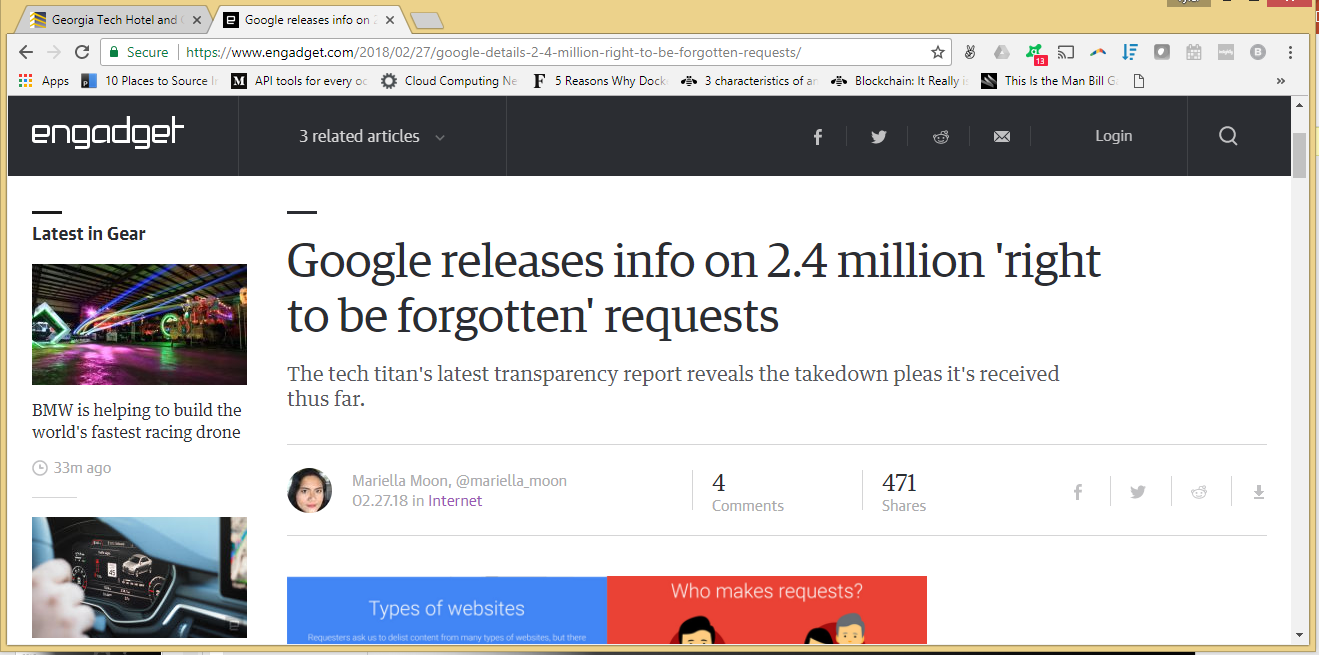The image is a screen capture of a website with two browser tabs visible in the upper left corner. The first tab, with a grey background, is labeled "Georgia Tech Hotel and." The second tab, colored white and currently active, reads "Google releases info." The webpage under the active tab belongs to the website https://www.ngadget.com. 

A black horizontal frame runs across the top of the webpage, with "Ngadget" written in white on it. This frame also indicates the presence of "Three related articles." In the main body of the webpage, a large headline prominently displays the text "Google releases info on 2.4 million right-to-be-forgotten requests" in black on a white background.